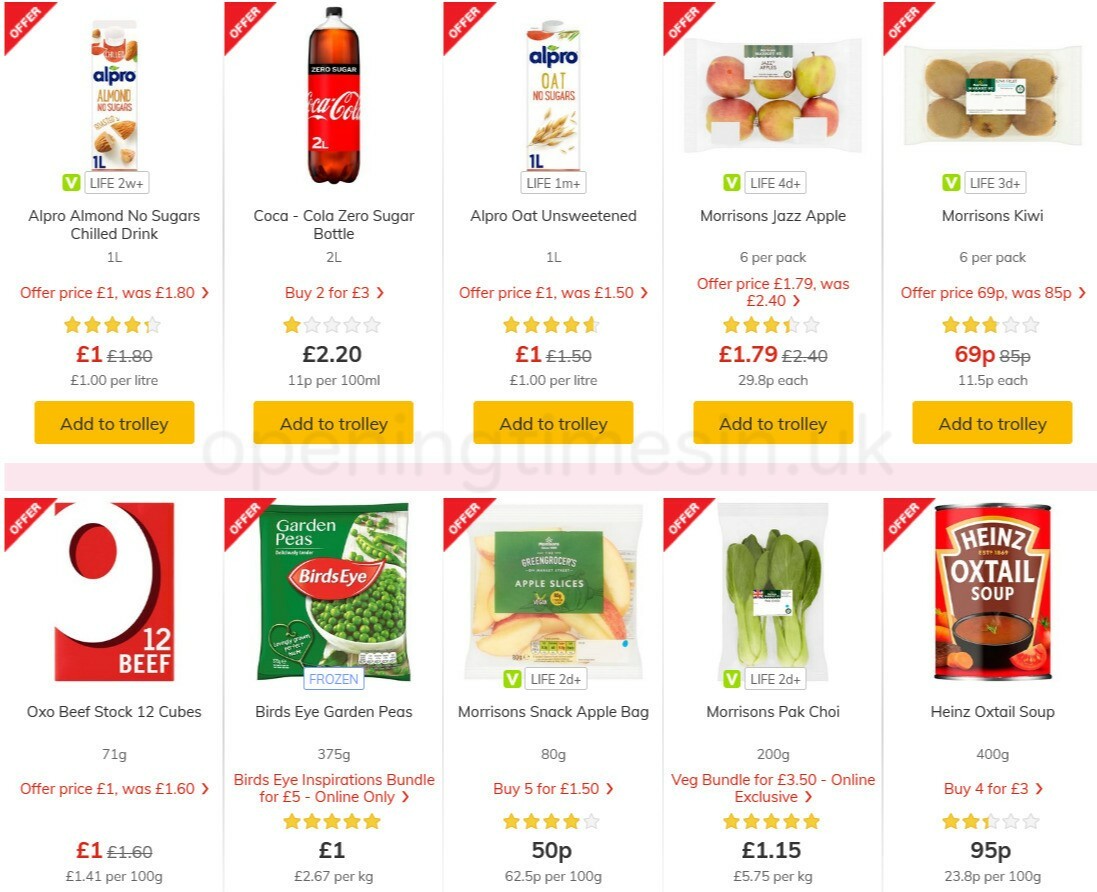On this website, users can collect a variety of offers on different products. Among the featured items, you can choose from a selection of drinks: an almond no sugars chilled drink (1 liter), a Coca-Cola Zero (2 liter bottle), and an all oat unsweetened drink (1 liter). For fruit lovers, there's Morrison's Jazz Apple six-pack and Morrison's Kiwi six-pack.

Moving to the second row, you have Oxo Beef Stock with 12 cubes, perfect for making beef bouillon. Right next to it, you'll find Birdseye's Garden Peas, and beside that, a convenient Morrison's Snack Apple bag with pre-sliced apples. Additionally, Morrison's Pak Choy comes neatly packaged in a bag. To round off the selection, there's Heinz Oxtail Soup available.

The prices for these items range from a high of £2.20 to a low of 50 pence for the apples, providing a variety of affordable choices for customers.